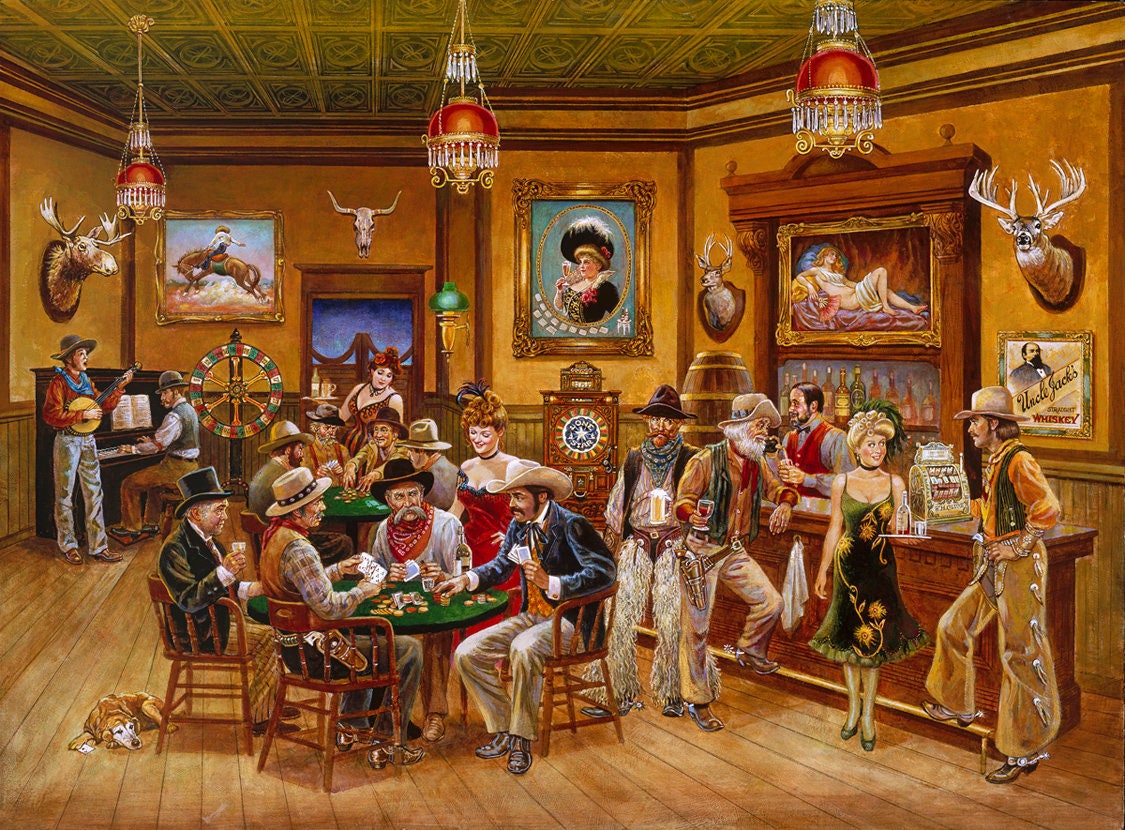The artwork depicts a lively, detailed scene set in an old-time Western saloon. The indoor setting features walls of tan wooden color adorned with framed portraits, two elk heads, an elk skull, and a moose head. Centered in the room, a green table is surrounded by four cowboy-hatted men engaged in a poker game, all seated on brown wooden chairs. The man closest to a yellow dog with a white face, black eyes, and black nose lays in the left corner, wears a green jacket and a black hat, holding something in his right hand. In the background, the bar area showcases a bartender serving drinks to several patrons, including two men leaning against the bar and a woman holding a drink. A piano player and a banjo player are situated on the left side, contributing to the lively atmosphere. Another card game is ongoing in the background. The overall scene is vividly captured, evoking a clear and bright Western ambiance richly detailed with various characters and activities.